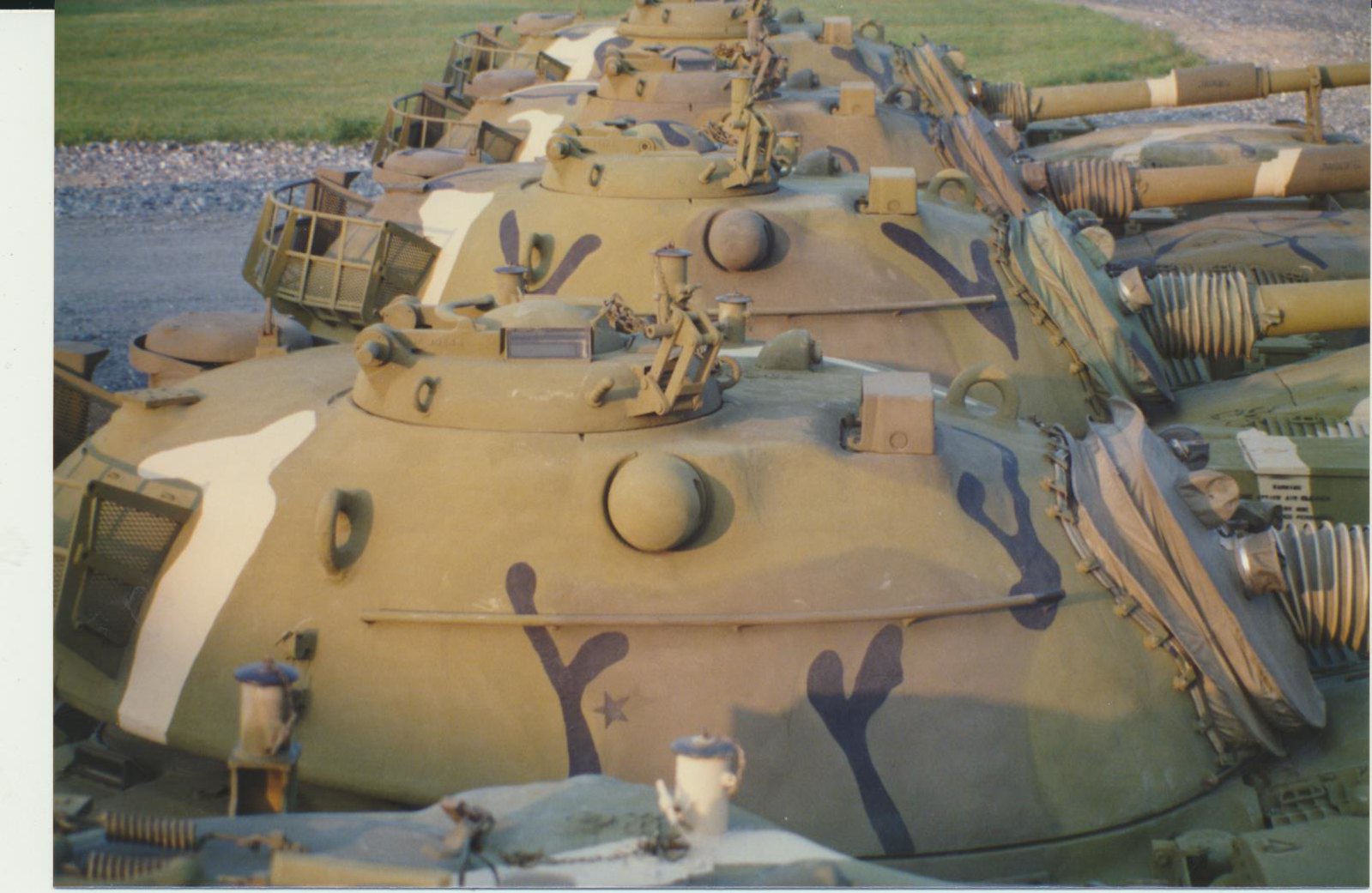This detailed color photograph captures four large military tanks lined up in a landscape orientation. The tanks, painted in a light brown and grey camouflage pattern with some black patterning, have their barrels pointing towards the left side of the image. Each tank features a prominent, dome-shaped top with a hatch and a visible cannon, extending outwards. A black star is painted near the bottom on the side of the front tank. These tanks are arranged in a line from the foreground, receding into the background, side on. In the backdrop, you can see a gravel road and patches of green grass. There are no people, animals, or additional structures present in this outdoor scene, emphasizing the stark, solitary arrangement of the military machinery against the natural landscape.